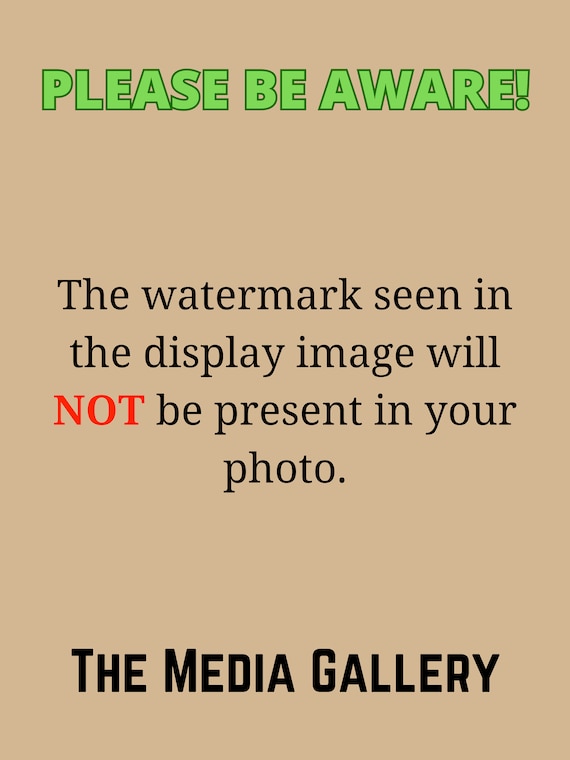This is an informative graphic, resembling an internet poster seen on websites like DeviantArt. It features a tan background designed in the format of a sign. At the very top, in striking lime green text with an exclamation point, it reads, "Please be aware!" Centrally aligned, in bold black text, it states, "The watermark seen in the display image will," with the word "NOT" emphasized in large red letters, "be present in your photo." At the bottom of the image, in prominent bold black lettering, it declares "the media gallery." The image is edge-to-edge with no watermarks, despite addressing watermark usage for displayed images on the site, clearly communicating that the visible watermark in gallery images will not appear in downloaded or purchased photos.